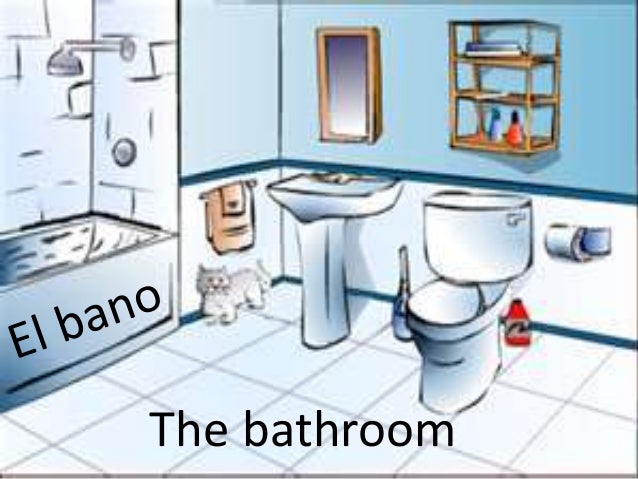The image depicts a cartoonish drawing of a bathroom interior designed with a blend of light blue, white, and gray colors. The floor is covered with bluish-white tiles. On the left, there is a bathtub featuring the text "El Baño" in black. Above the bathtub is a shower faucet. Moving forward, a cat is seen near the wall beneath two hanging towels on a towel rack. The bathroom features a pedestal sink with a square basin and a square mirror mounted above it. To the right of the sink, a white toilet is positioned with a toilet brush on its left and a toilet bowl cleaner on its right. To the right of the toilet hangs a roll of toilet paper on the wall. Above the toilet, there is a square shelf holding various items such as books and bottle cleaners. The image includes elements such as a red liquid bottle and cleaners, with "The Bathroom" also written across the front, emphasizing it might be a tool for teaching Spanish to English or vice versa.